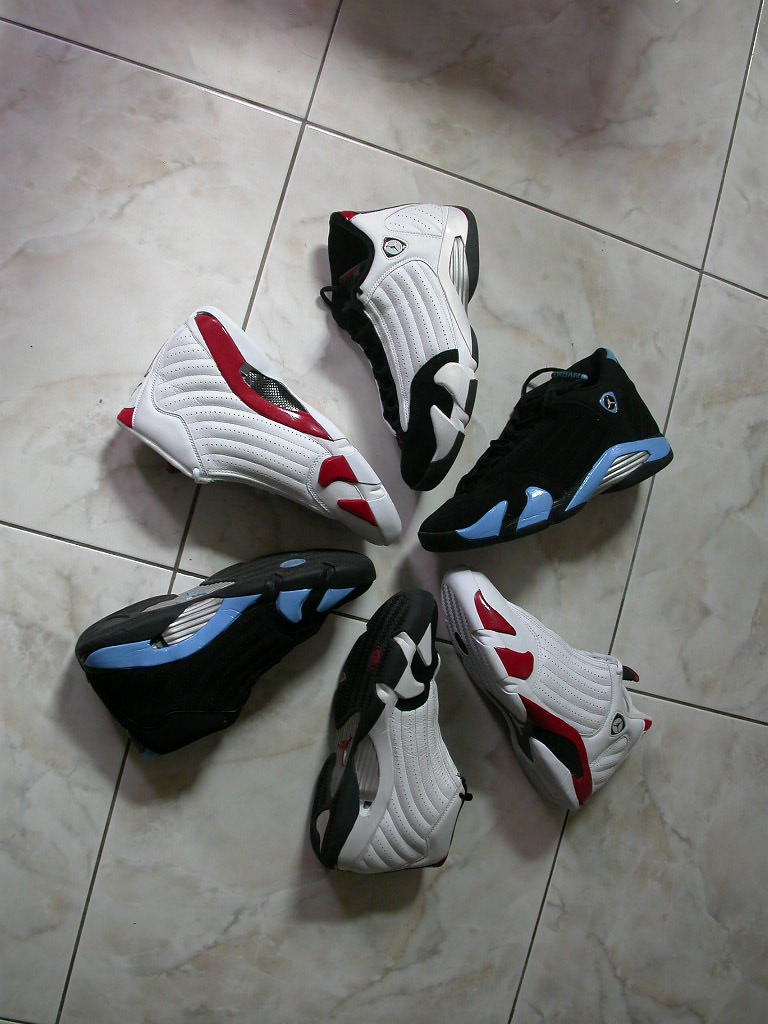In the image, a detailed view from above reveals a large square-tiled floor, possibly made of white or light grayish stone or marble. Centered on the tiles, six medium high-top athletic basketball shoes are artfully arranged in a circular, pinwheel-like pattern, toes pointing inward. The shoes, likely branded by Puma, appear to be children's tennis shoes. Each pair of shoes is distinct in color and arrangement: 

- At the 12 o'clock position, a predominantly white shoe with black lines.
- Moving clockwise to 2 o'clock, a black shoe with blue soles.
- At 4 o'clock, a white shoe featuring red details.
- At 6 o'clock, another white shoe, this time with black soles.
- At 8 o'clock, a black shoe with blue accents.
- Finally, at 10 o'clock, a white shoe with red accents.

There are discernible shadows cast on the floor, hinting at the presence of overhead lighting and suggesting the image may have been taken in a kitchen.